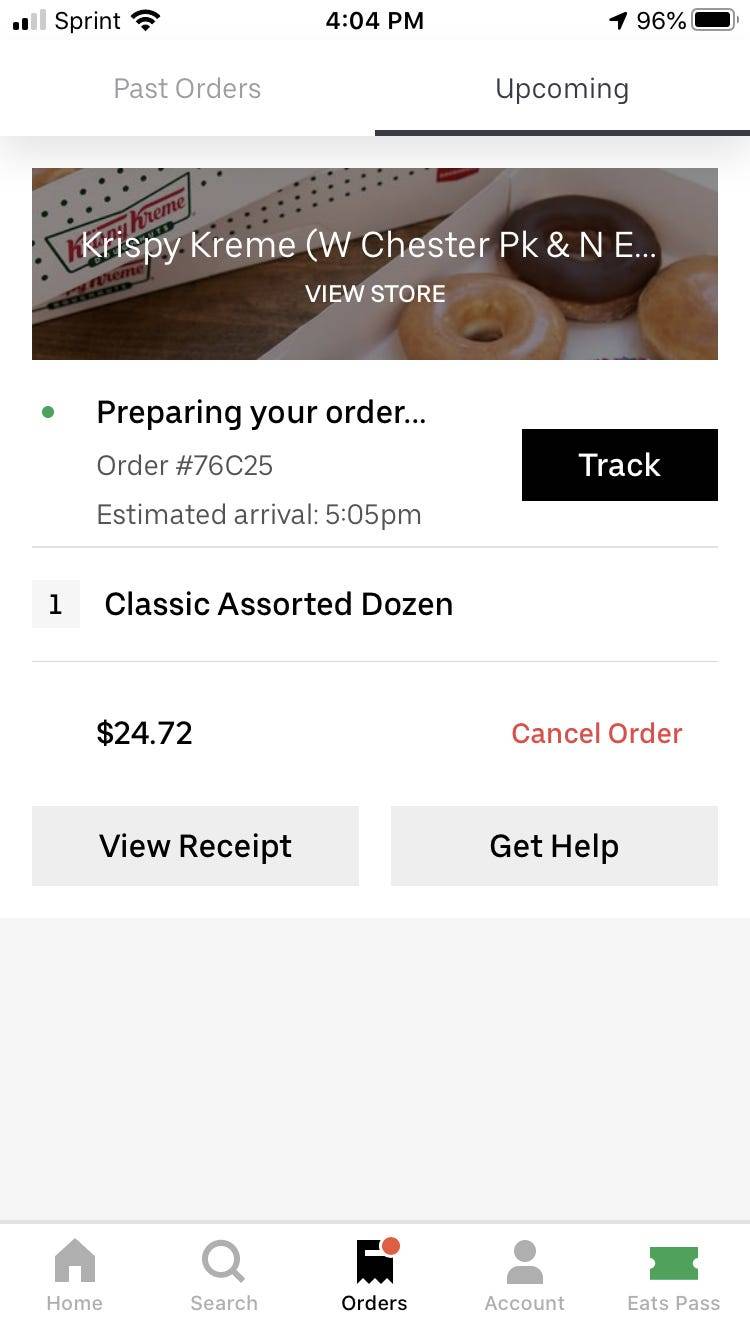A detailed screenshot of the Uber Eats app reveals various elements of an ongoing order. In the top left corner, the user has Sprint as their mobile carrier, showing two bars of signal strength and a Wi-Fi connection. It is 4:04 p.m., and the top right corner discloses a 96% battery level. Below the app's header, the screen is divided into "Past Orders" and "Upcoming," with the "Upcoming" tab currently selected.

A photograph displays two glazed donuts and a chocolate donut inside a Krispy Kreme box. The location is partially visible in parentheses as "Westchester Park and Northeast..." Below the image, the status reads "Preparing Your Order," indicated by a green dot and an ellipsis. The order number is 76025 with an estimated arrival time of 5:05 p.m. A "Track" button is available next to this information.

The order summary includes "One Classic Assorted Donut Dozen" priced at $24.72. Below this, options to "Cancel Order," "View Receipt," and "Get Help" are provided. The navigation bar at the bottom of the screen features a "Home" button, a "Search" button, an "Orders" button (highlighted to show it's the current screen), an "Account" button, and an "Eats Pass" button.